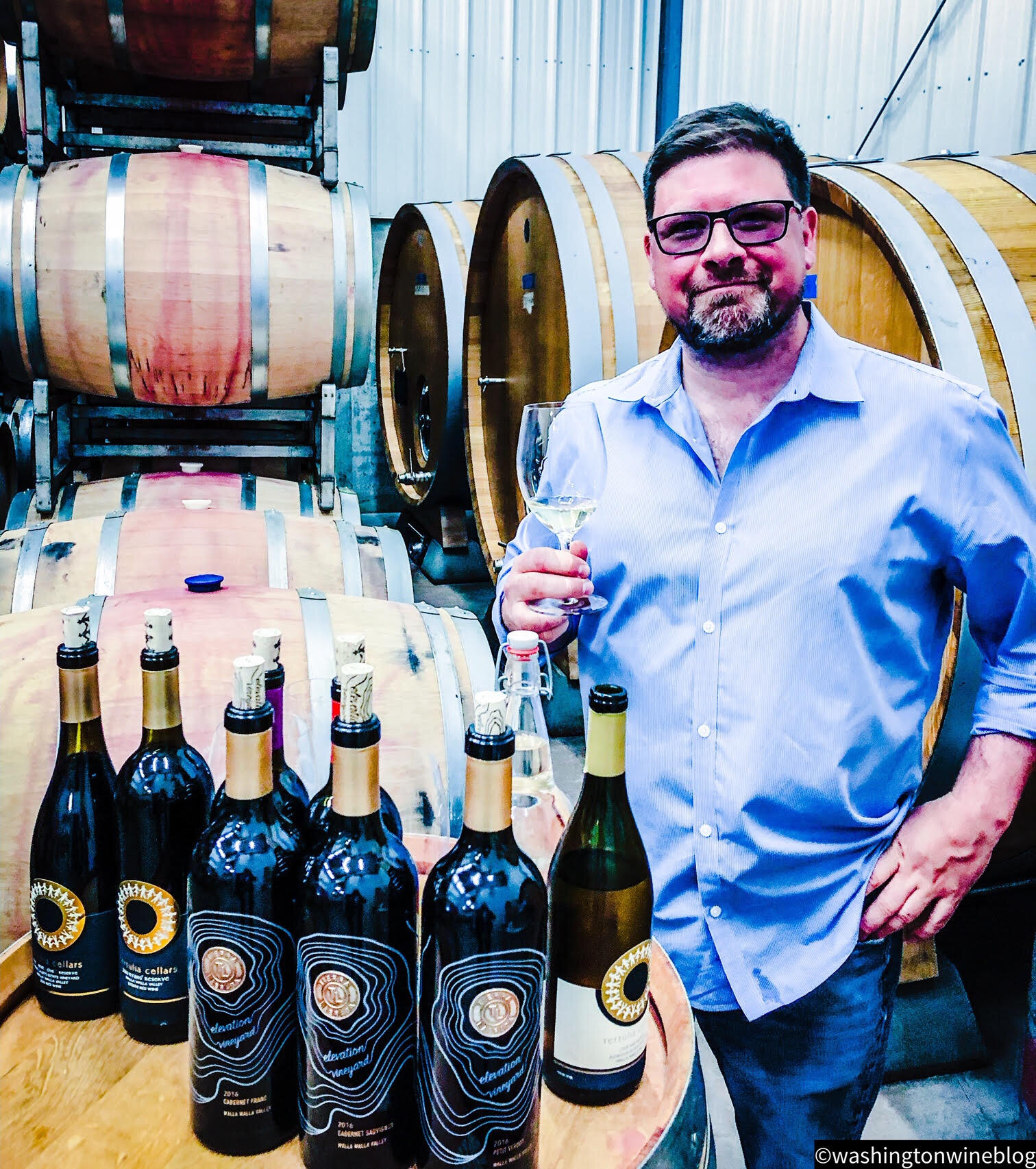In this color photograph, a cheerful man stands in a distillery, evidently enjoying his surroundings. He has short dark hair, a salt-and-pepper beard, and wears black-framed glasses with a slight tint to the lenses. His facial expression is pleased, with a closed-mouth smile. He is casually dressed in a blue button-down shirt with the collar slightly open and stonewashed blue jeans. With his right hand, he holds a wine glass, partially filled with what appears to be wine, raised in a toasting gesture towards the camera, while his left hand rests on his hip. The background features numerous wooden wine barrels, suggesting a wine-tasting room. In front of him, bottles of wine are arranged atop one of the barrels. Notably, there are six bottles—three dark blue with a concentric pattern, and another three with a round donut-like pattern—indicating a variety of wines. At the bottom right of the image, the inscription reads, "Copyright Washington Wine Blog."